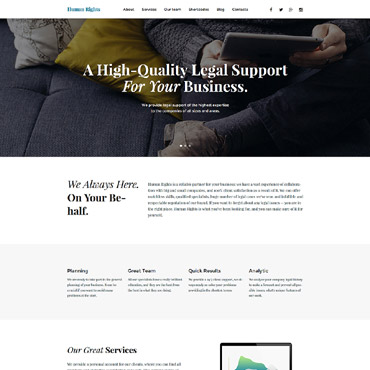In the center of the image, there is a neatly designed box featuring a dark blue couch adorned with yellow and white throw pillows. A person is seated on the couch, dressed in a long gray sweater, pants, and brown shoes, holding either an iPad or a phone. Central to the image is the text "High-Quality Legal Support for Your Business," accompanied by the phrase "We're always here on your behalf" situated just below and slightly to the left. To the right, a small paragraph of black text provides additional information. Below this section, the image is divided into four areas, highlighting "Quick Results" and "Analytics" among the choices. At the bottom left corner, a bold black text reads "Our Great Services." To the right, a layered square design features a black top, a white center, and a green color within. In the upper right corner, there are small icons for sharing on Facebook (an "F") and Twitter (a bird).